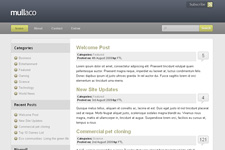The website image for the company Mulaco (spelled M-U-L-L-A-C-O) is notably blurry, making some text difficult to decipher. At the top of the page, a wide, dark gray ribbon spans across, featuring the company’s name "mulaco" in lowercase white text situated in the left-hand corner. Directly below this, a thinner, light gray ribbon extends horizontally across the page. On the far left of this ribbon is a yellow button with unreadable black text inside, followed by additional white text to its right. Positioned on the far right is a white search bar.

Below these ribbons, the background transitions to a light gray. Dominating this section is a smaller white box, the left third of which contains a vertically running, wide light gray ribbon. At the top of this vertical ribbon, "Categories" is written in black text. Below, there are several indiscernible terms listed in light gray text in a vertical format. A secondary category label appears below in black text, likely reading "Recent Something" (although the remaining text is not clear), followed by more unreadable light gray text entries.